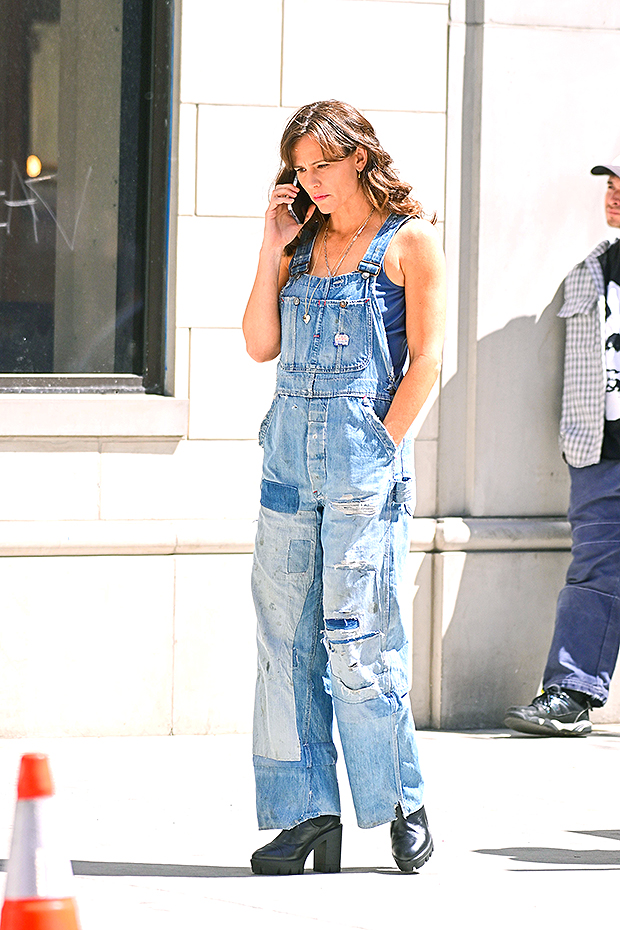The image is a vertically rectangular, full-color photograph taken outdoors on a sunny day. The main focus of the photo is a young Caucasian woman with wavy, shoulder-length brown hair, presumed to be actress Jennifer Garner. She is standing on a sidewalk, facing slightly to the left and towards the camera, with a cell phone held up to her right ear by her left hand. Jennifer is dressed in a blue sleeveless top under a pair of lighter blue jean overalls. Her left hand is casually tucked into her pocket, and she is wearing high-heeled black boots. A silver necklace adorns her neck.

Behind Jennifer, the backdrop consists of a white cinder block building with a black window framed in white at the upper left corner. On the right edge of the photograph, partially visible, is a young Caucasian man leaning against the building. He is wearing a black and white checkered collared shirt over a black t-shirt with a white logo, complemented by blue jeans, dark shoes, and a baseball cap.

In the foreground, on the lower left-hand corner of the image, there is an orange and white traffic cone. The overall scene provides a casual yet detailed slice of everyday urban life.